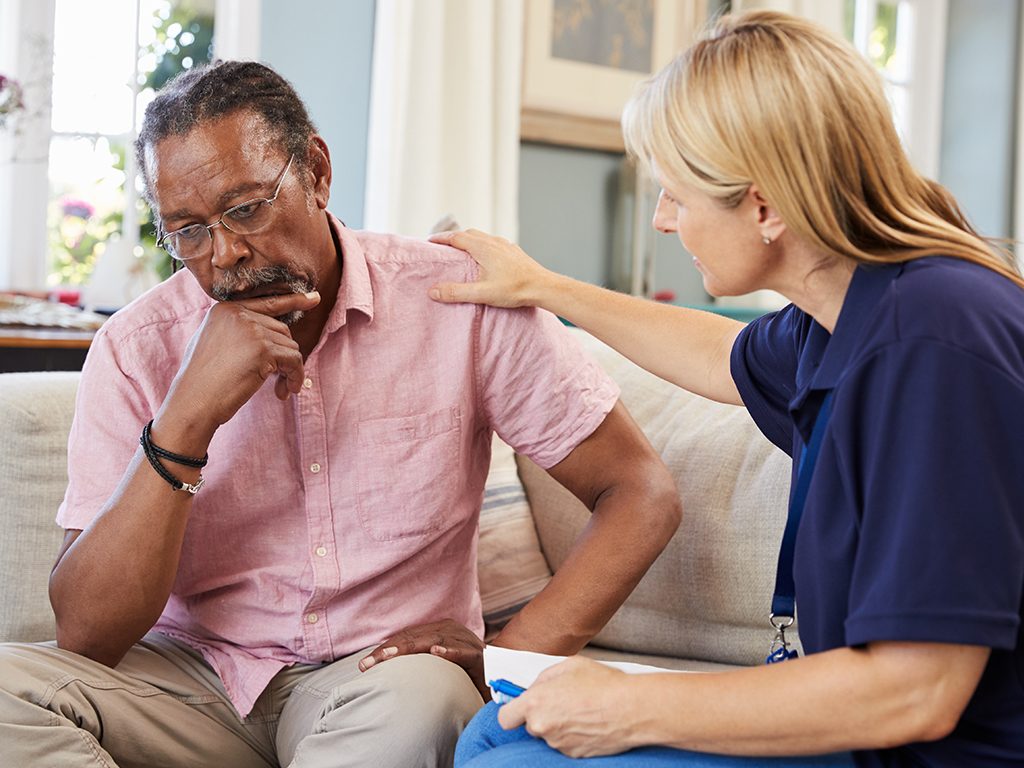In a cozy living room setting with blue and white decor, complete with white curtains, a portrait on the wall, and a table adorned with reddish blooms and green foliage, two individuals are seated on a cream-colored linen couch. The focus is on a contemplative black gentleman, who sits pensively with his right elbow resting on his leg and his hand positioned just below his lower lip. He wears a pink short-sleeve button-up shirt, taupe-gray pants, a black braided bracelet on his right wrist, and wire-rim silver glasses that accentuate his thoughtful gaze downward. Beside him is a sympathetic blonde lady, who appears to be a professional, indicated by the name lanyard around her neck and the papers and pen she holds. Dressed in a dark blue polo shirt, she extends a comforting right hand to rest on the gentleman’s left shoulder, conveying support and understanding during what seems to be a difficult decision-making moment.